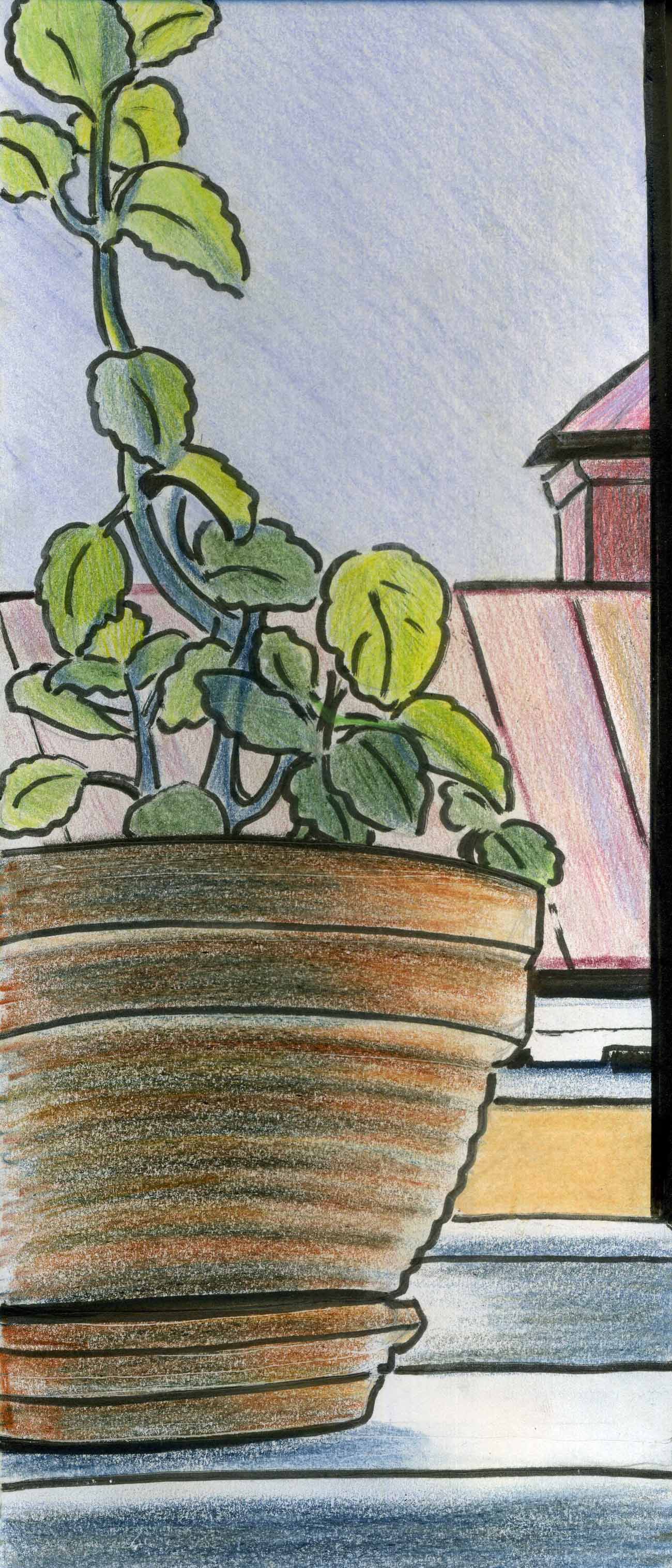This color illustration, rendered with black marker and colored pencils, portrays a potted plant on a windowsill. The plant is housed in a brown pot that rests on a matching drainage saucer, both placed securely on a white window ledge. The plant itself is tall and verdant, featuring lush green leaves but no flowers. In the background, a building with a visible roof and chimney is seen under a clear blue sky. The vertical orientation of the image accentuates the height of the plant and the depth of the background. There are no inscriptions, human figures, billboards, signs, or animals depicted in this detailed and tranquil scene.